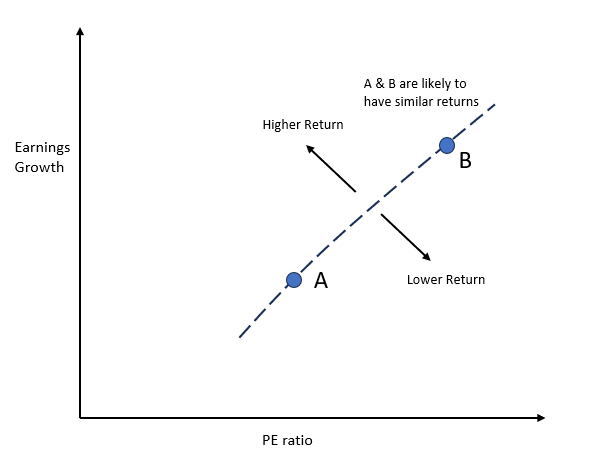A minimalistic graph is depicted on a plain white background, illustrating the relationship between the Price to Earnings (PE) ratio and earnings growth, which are significant metrics in the context of investing and stocks. The x-axis represents the PE ratio while the y-axis indicates earnings growth. The graph features two labeled data points: 'A' positioned in the bottom-left quadrant and 'B' situated in the top-right quadrant. A dotted line connects these points, forming an upward diagonal trajectory from left to right, signifying increment.

Annotations next to the dotted line suggest that points 'A' and 'B' are likely to yield similar returns. Arrows extending from both ends of the dashed line indicate that movement along the line implies varying returns, with one side denoted as 'higher return' and the other as 'lower return'. This visual representation underscores the general relationship that as the PE ratio increases, earnings growth also rises, highlighting a common trend in stock investment evaluation.